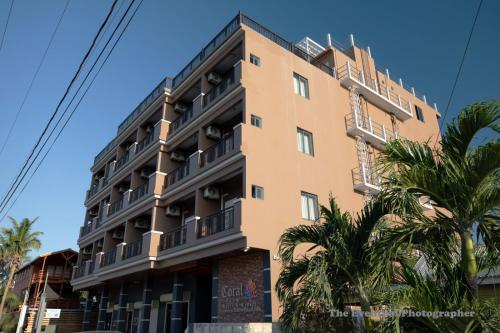The photograph captures a detailed view of a beige-brown, five-story, cubic building during the daytime. The image shows the right side of the building prominently, where three windows line the side and a white fire escape ladder is attached. The bottom left corner of the image reveals part of another building, likely wooden, accompanied by a palm tree. Dominating the lower right corner are tall banana leaf plants and additional palm trees. 

The front of the building features three balconies and a recessed base supported by black columns. A sign on the building reads "coral," although the second word is not entirely clear. At the bottom right of the image, barely legible text appears to mention "photographer," but the preceding text is blurry. 

Above the building, four electric lines stretch diagonally from the top-left to the center left of the image, set against a backdrop of a blue sky. The scene is detailed with architectural elements, greenery, and utility lines, providing a comprehensive view of the urban setting.